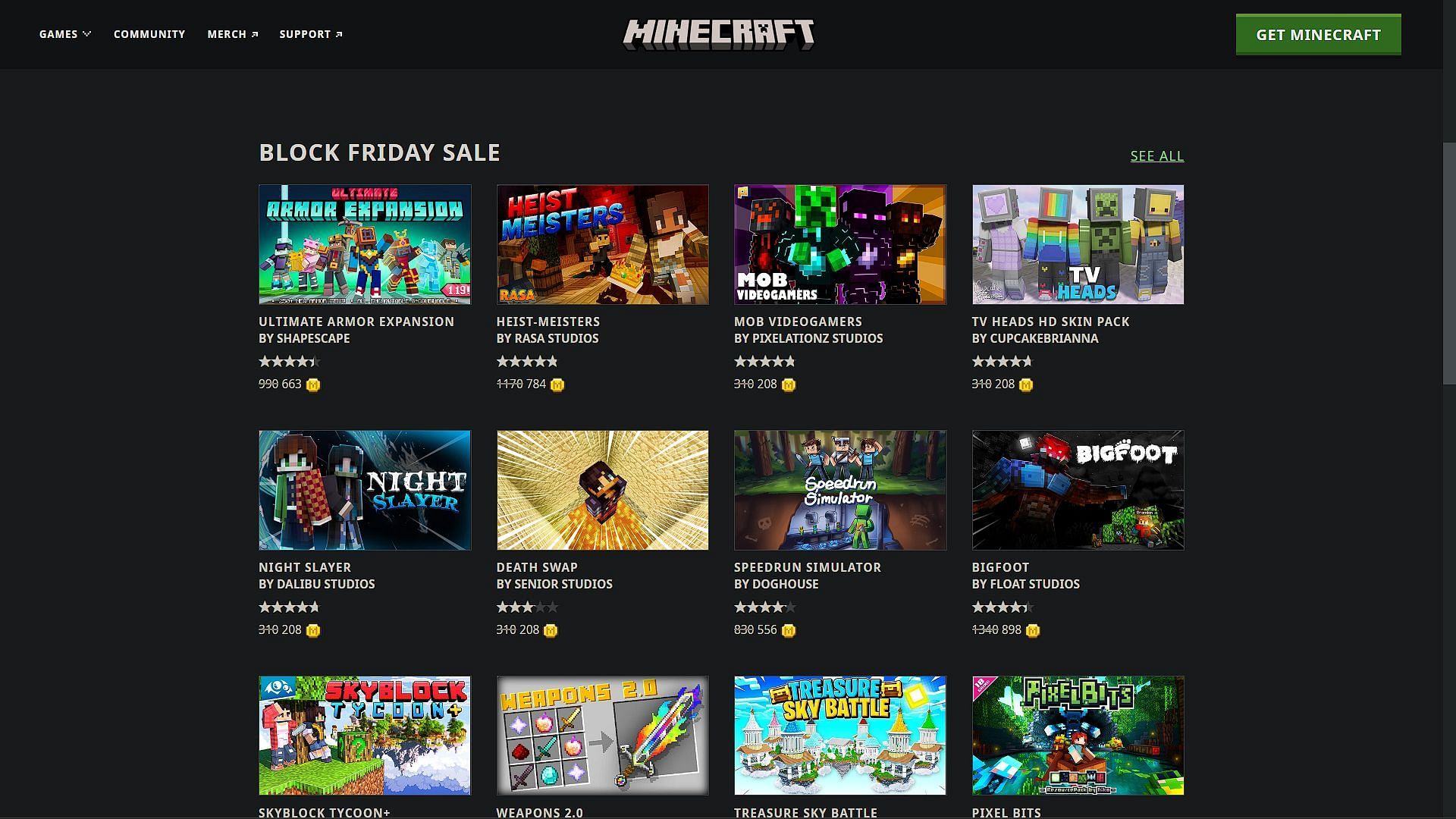This screenshot is taken from a computer or laptop monitor displaying a predominantly black background. In the upper left-hand corner, there are four white labels organized vertically: "Games," "Community," "Merch," and "Support." Centralized in the middle of the screen, large bold white letters spell out "Minecraft." Towards the top right corner is a rectangular green button with white text that reads "Get Minecraft."

Directly below, on the left side, there is a bold white heading, "Block Friday Sale," clearly a play on "Black Friday Sale." Underneath this heading are three rows of four thumbnails each, showcasing various Minecraft expansions and items available during the sale.

In the first row of thumbnails:
1. **Ultimate Armor Expansion**
2. **Heist Meisters**
3. **Mob Video Gamers**
4. **TV Heads HD Skin Pack**

The second row offers more in-game content:
1. **Night Slayer by Dalibu Studios**
2. **Death Swap**
3. **Speedrun Simulator**
4. **Bigfoot**

The final row features different game-related content:
1. **Skyblock Tycoon**
2. **Weapons 2.0**
3. **Treasure Sky Battle**
4. **Pixel Bits**

Each thumbnail appears to be a vibrant screengrab or cover image from within the Minecraft universe.